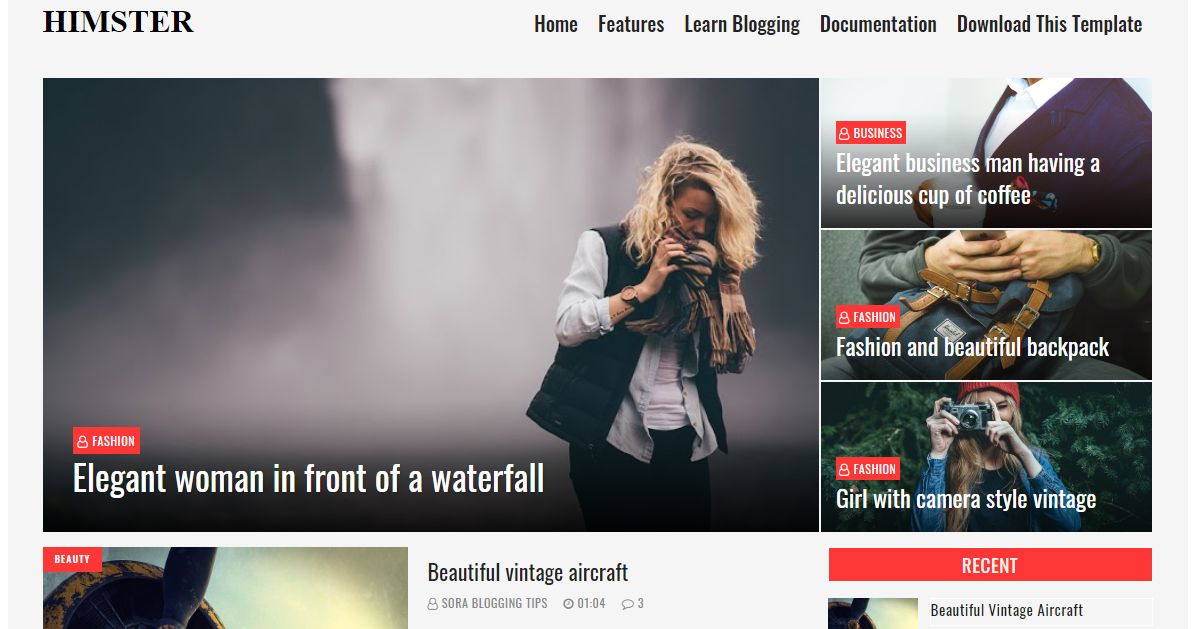The image is a horizontally rectangular screenshot of the upper portion of a website, featuring a predominantly light gray background. At the very top left corner of the image, "HIMSTER" is written in all capital letters. To the right of "HIMSTER," there is a navigation menu including options for "Home," "Features," "Learn Blogging," "Documentation," and "Download This Template."

In the right half of the frame, there are three vertically stacked, horizontally rectangular images. The top image depicts an elegant businessman enjoying a cup of coffee. The center image showcases a fashionable, beautiful backpack. The bottom image features a girl with a vintage-style camera.

On the left side of the frame, there is a large, horizontally rectangular image with a grayish background. This image shows a person with long blonde hair looking down towards the bottom right corner. They are dressed in a white undershirt with an unbuttoned long-sleeve shirt layered over it and a black vest. In the bottom left corner of this image, the text reads "Elegant woman in front of a waterfall."